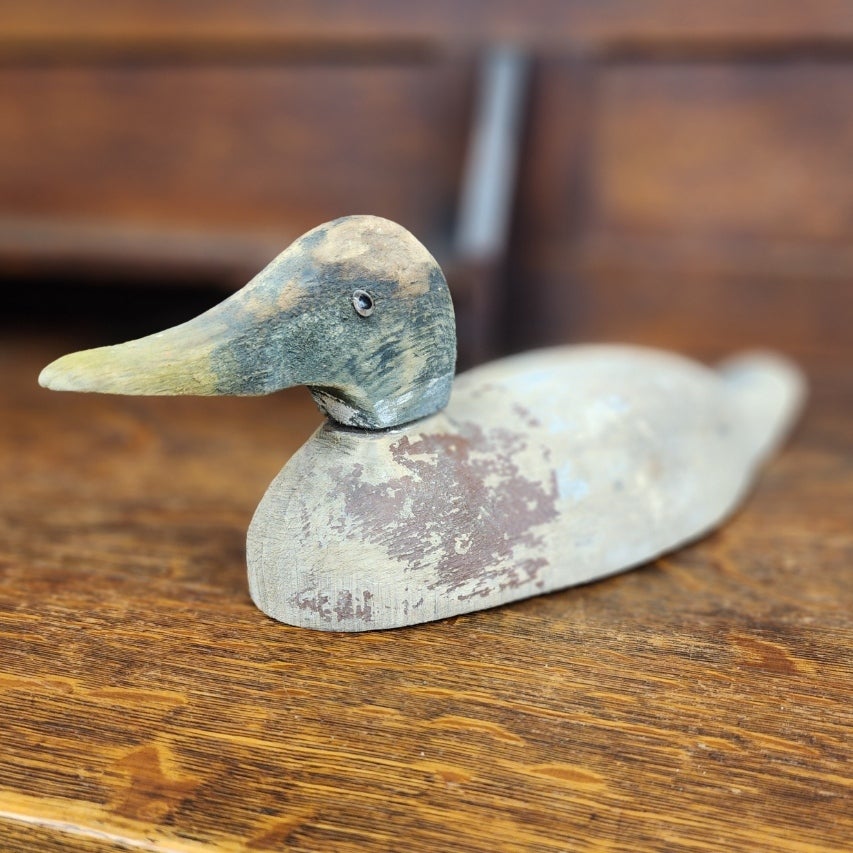This is a detailed photo of an antique carved wooden duck, distinguished by its heavily worn and weathered appearance. The duck, likely meant to resemble a mallard, exhibits a simplified shape with a yellow beak and a faded black spot for an eye. Once vibrant with paint, the body now reveals mere patches of what might have been black or green, blending with the prevailing gray, dull reddish-brown hues, and the exposed old wood. The head is still attached to a base that hints at having been red at one point. This aged artifact rests on a newer wooden surface, possibly a table or floor, and the background—featuring an indistinct wooden cabinet or similar brown wooden item—remains out of focus, further emphasizing the duck's vintage charm.